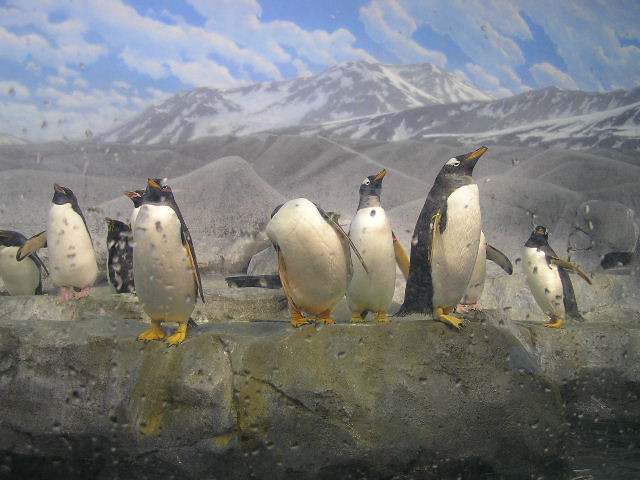A photograph captures a group of approximately nine penguins standing at the edge of a gray, rocky cliff. They have distinctive white bellies, black backs, and black wings with orange feet. The penguins, with small patches of white around their eyes, have orange beaks and are mostly looking upwards with their wings spread. The backdrop features a majestic mountain range with snow-capped peaks that descend into gray rock formations, resembling a triangle in shape. Above, the sky is bright blue, dotted with fluffy white cumulus clouds. The daylight and detailed depictions suggest the image was taken during the day, and there seems to be water droplets on the lens, indicating rainfall.